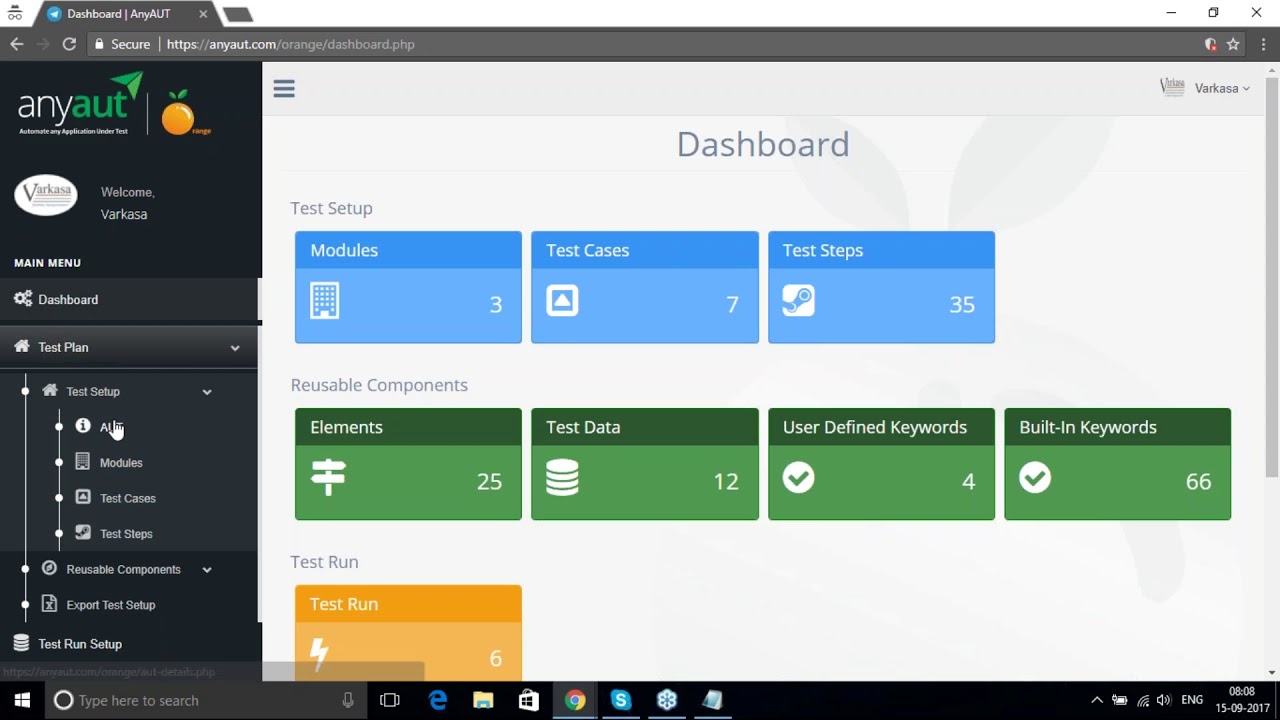This is a descriptive caption for the given screenshot:

---

The screenshot is from a platform called "AnyAught" (spelled A-N-Y-A-U-T), featuring a green paper airplane icon adjacent to the title. To the right of the title, there is an orange fruit illustration with two green leaves. Below this, the text "Welcome for VARCASA" is displayed. The left side of the webpage houses a black vertical main menu bar with several options. The main menu options listed are: "Main Menu," "Dashboard," "Test Plan" (which expands to "Test Setup" and another obscured word), "Modules," "Test Cases," "Test Steps," followed by "Reusable Components," "Expert Test Setup," and "Test Run Setup."

On the right-hand side, which comprises approximately three-quarters of the page and has a white background, the top navigation includes a three-bar menu button and "VARCASA" accompanied by a down arrow on the right. The main body of the page showcases several colored rectangles. There are three blue rectangles labeled "Modules," "Test Cases," and "Test Steps." Below these, four green rectangles are labeled "Reusable Components," "Elements," "Test Data," "User-Defined Keywords," and "Built-In Keywords." At the bottom, there is an orange rectangle labeled "Test Run."

---

This caption offers comprehensive details about the visual elements and layout of the page.